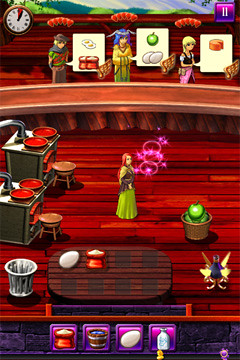This is a detailed screenshot from a mobile video game showcasing a vibrant kitchen scene. At the center of the image, a female character, identifiable by her red hair and green dress with a black apron, stands on a platform resembling a redwood floor. She is engaged in a magical activity, with pink circles and pink stars emanating from her, indicating a spell or special action. Directly behind her are two stoves equipped with pots of red sauce, possibly tomato sauce, along with stools in front of each stove and exhaust pipes visible in the background. To the left of the stoves, there's a wastebasket and a table, while on the right, a bucket filled with a green liquid and a green apple is seen.

The top of the screen features three characters beside individual signs displaying different food products. One male character wears a round hat and a green-red shirt, associated with images of eggs and red pots. A blue-haired woman is depicted with icons of eggs and a green apple. Lastly, a blonde-haired maiden with a light blue top and pink sash is shown next to a sign with either a cake slice or a round cheese with a slice missing.

At the very top-left corner, a clock is partially visible, likely indicating the remaining time for task completion in the game. The lower part of the screen showcases a purple bar with four purple squares containing various objects, including an egg and a bag of flour or sugar.